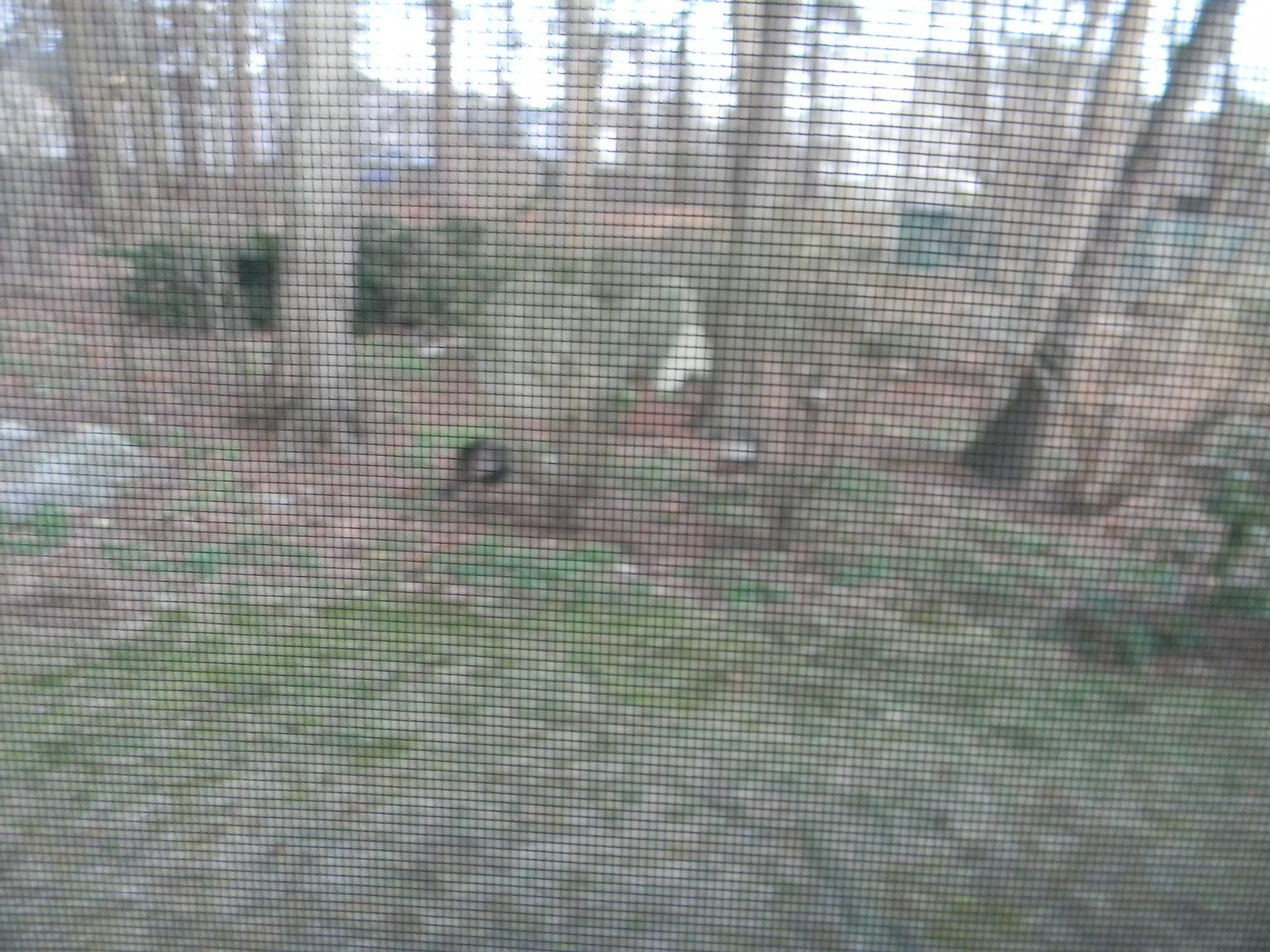The image captures a scene viewed through the fine, black grating of a netted door or window. The grid-like pattern of the wires creates small, square compartments that partially obscure the background. Beyond the grating, the ground appears predominantly green, interspersed with areas of dried foliage. Scattered leaves are visible, adding texture to the scene. Trees with thick bark and thin trunks stand tall, some extending out of view. In the distance, a lush green bush provides a burst of verdant color. Although unclear, there is a possibility of an animal presence amidst the greenery. At the center of the scene, several boulder-like rocks protrude from the ground, adding a rugged, natural element to the landscape.